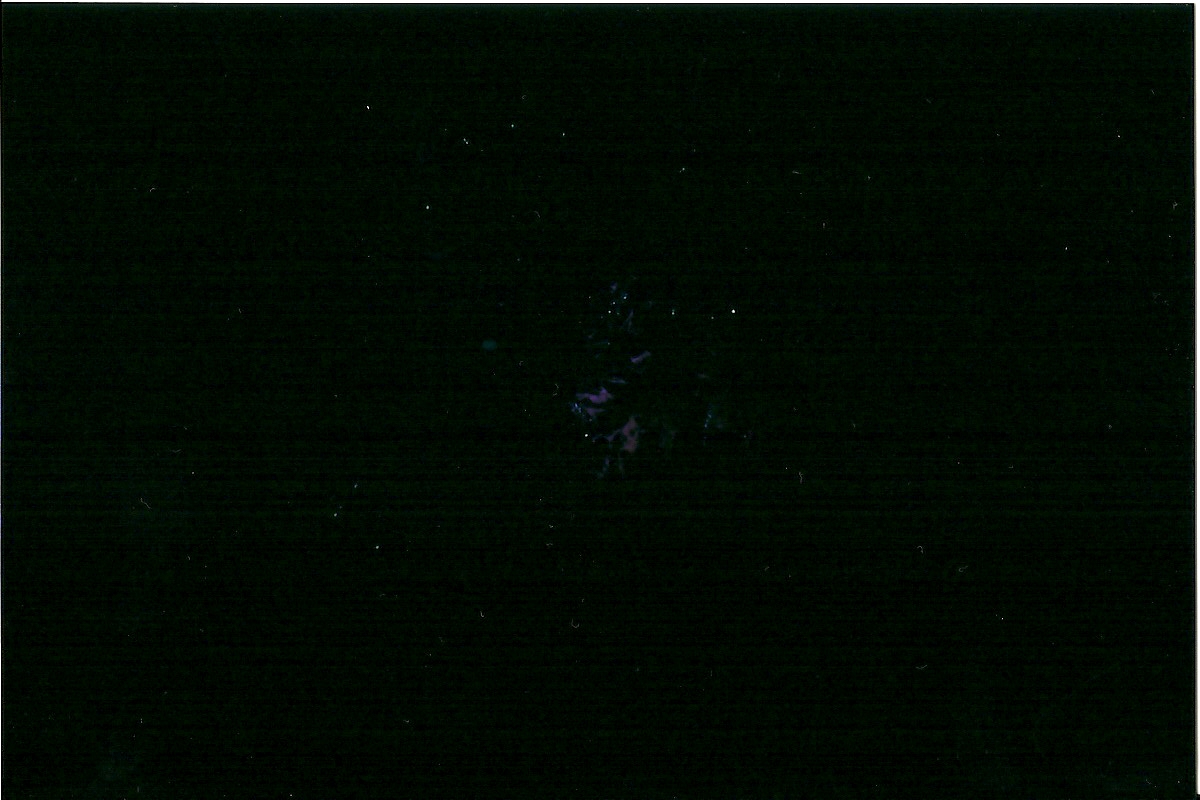This captivating photograph of outer space showcases a vast expanse of the night sky. The predominantly black backdrop is intermittently dotted with twinkling stars, evoking a sense of the infinite cosmos. In the central region of the image lies a faint, yet mesmerizing, distant galaxy, offering a glimpse into the wonders beyond our solar system. At the top of the photograph, a group of stars forms a potential constellation, adding to the celestial charm. On the center-left side, an intriguing arrangement of stars appears in an upside-down, tilted L shape, possibly part of another constellation. The overall composition of the image presents a breathtaking window into the mysteries of the universe.